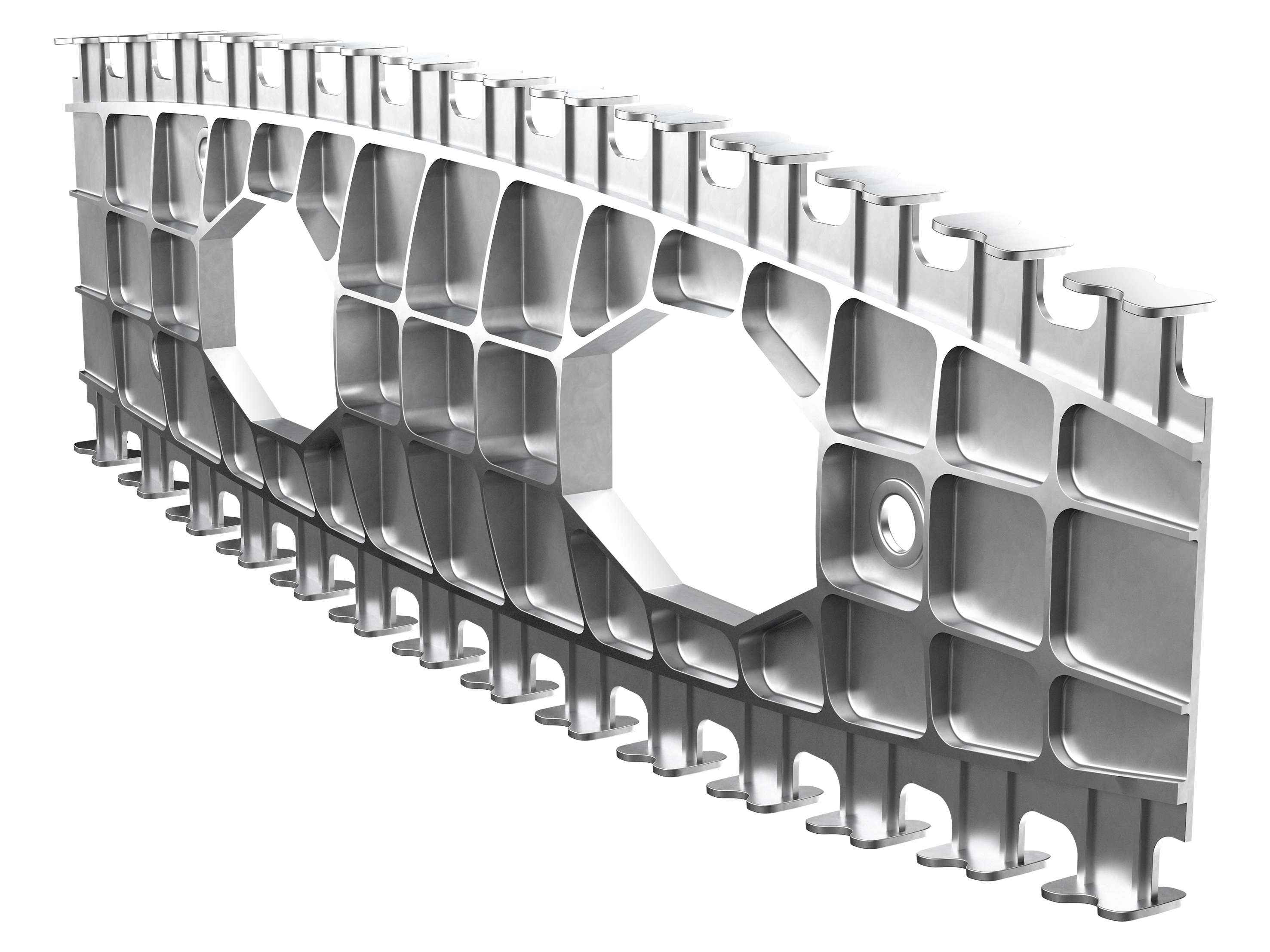This image depicts a computer-generated piece of metal that appears to be a part of a vehicle, possibly looking like a grill or license plate cover. The metal object is rectangular and features five horizontal rows. Notably, there are square-shaped indentations spanning the length of the piece. The center row is punctuated by two large octagon-shaped cutouts, one on the left and one on the right, which allow light to pass through, creating a white background. Additionally, on the right side adjacent to the octagon in the middle row, there's a small hole. The metal's shading transitions from lighter at the top to darker at the bottom. Along the top and bottom edges of the object are flat-topped rods that extend in diagonal lines. The piece stands on fourteen short legs, contributing to its structured and supported appearance.